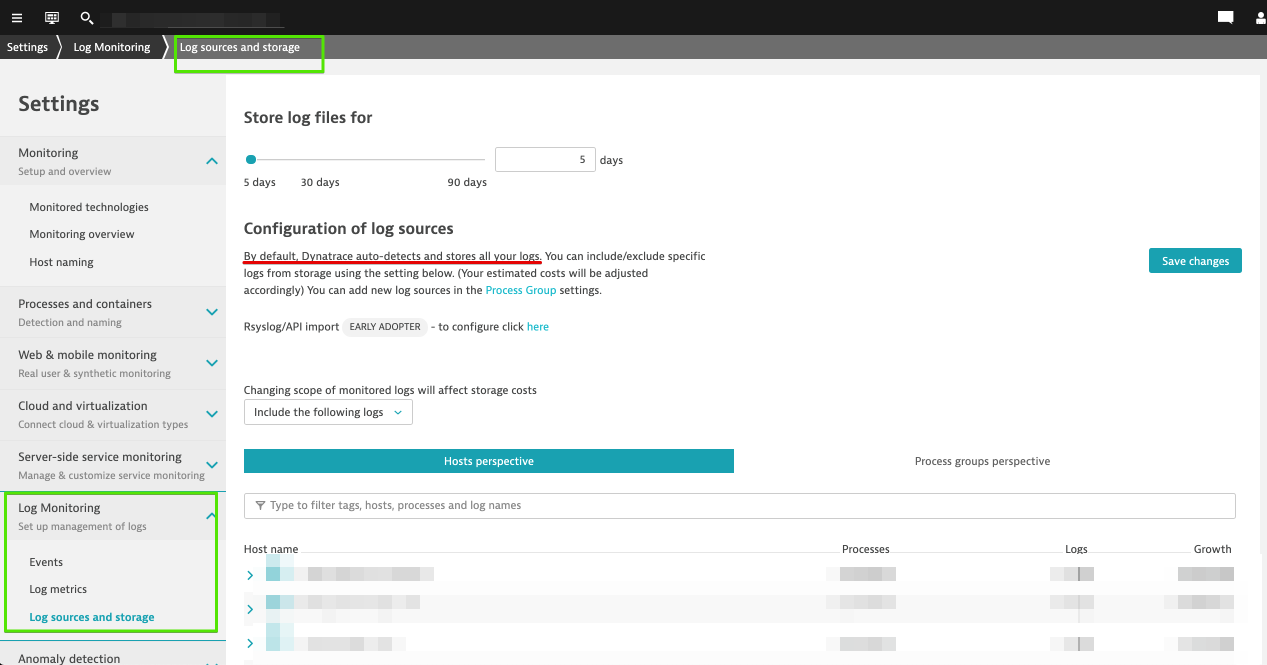The image showcases a settings page within a software application, specifically focusing on logging and monitoring configurations. On the left-hand side of the interface is a vertical menu under the overarching header "Settings." The top section of this menu is labeled "Monitoring," and it is expanded to reveal additional options including "Monitor Technologies," "Monitored Overview," and "Host Naming." 

Below the "Monitoring" section, there are four more collapsed sections with the fifth one expanded, labeled "Log Monitoring." Within this section, sub-options such as "Events," "Log Metrics," and "Log Sources and Storage" are visible.

The right side of the interface, taking up the main content area, is currently displaying the "Store Log Files" settings. It indicates that log files are set to be stored for a period of five days. Following this, the "Configuration of Log Sources" is detailed with an emphasized note in red: "By default, Dynatrace auto-detects and stores all your logs." 

This structured layout provides a comprehensive overview of available logging and monitoring settings, highlighting critical configurations for log file storage and source detection.